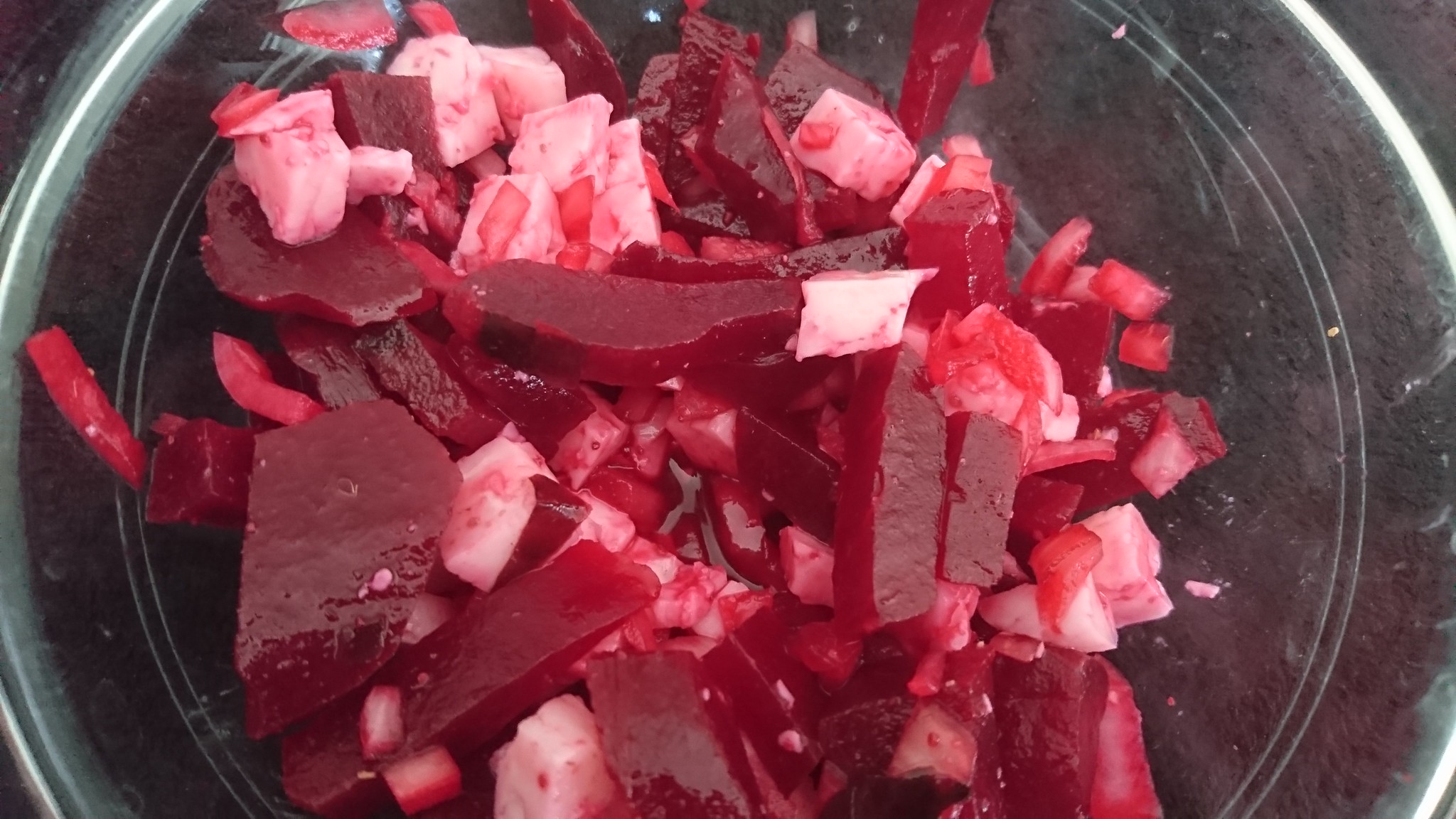The image portrays a super close-up view of a glass bowl placed on a dark, possibly black or brown, surface. Inside the bowl, there are various chunks of bright red, pink, and white substances. These chunks appear to have been broken or chopped into irregular, rectangular, and pointy bits. The predominant color is a vivid, blood-red, accompanied by pieces that are pink or white with a hint of red. The materials within the bowl could be food substances like cranberry sauce, possibly mixed with something resembling tofu or diced mayo, although some interpretations suggest they might be wax or plastic. The photo's angle is from above, providing a clear view of the vibrant, contrasting colors and the translucent nature of the glass container.